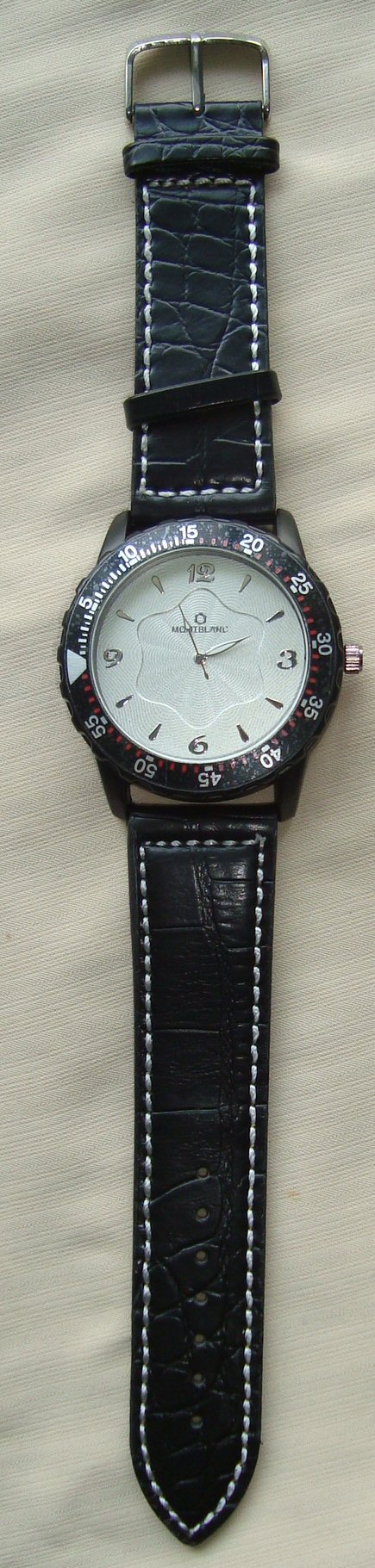The image showcases a wristwatch fully extended to display its entire length, including the loop, watch face, and metal connector for adjusting the fit. The background appears to be a fabric with a whitish, grayish, and tan hue, featuring very thin diagonal lines. At the top of the watch, there is a metal bar with a small clicker used for securing the watch around the wrist. Further down the upper half, there's a loop through which the leather material is threaded to tighten the watch. 

The watch face itself is white, encased in a black frame that marks intervals of five seconds. The dial features the numbers 12, 3, 6, and 9 at their respective positions, with dashes indicating the other hours. Minute and hour hands are also present. There are seven holes for adjusting the tightness of the wristwatch to ensure a proper fit.